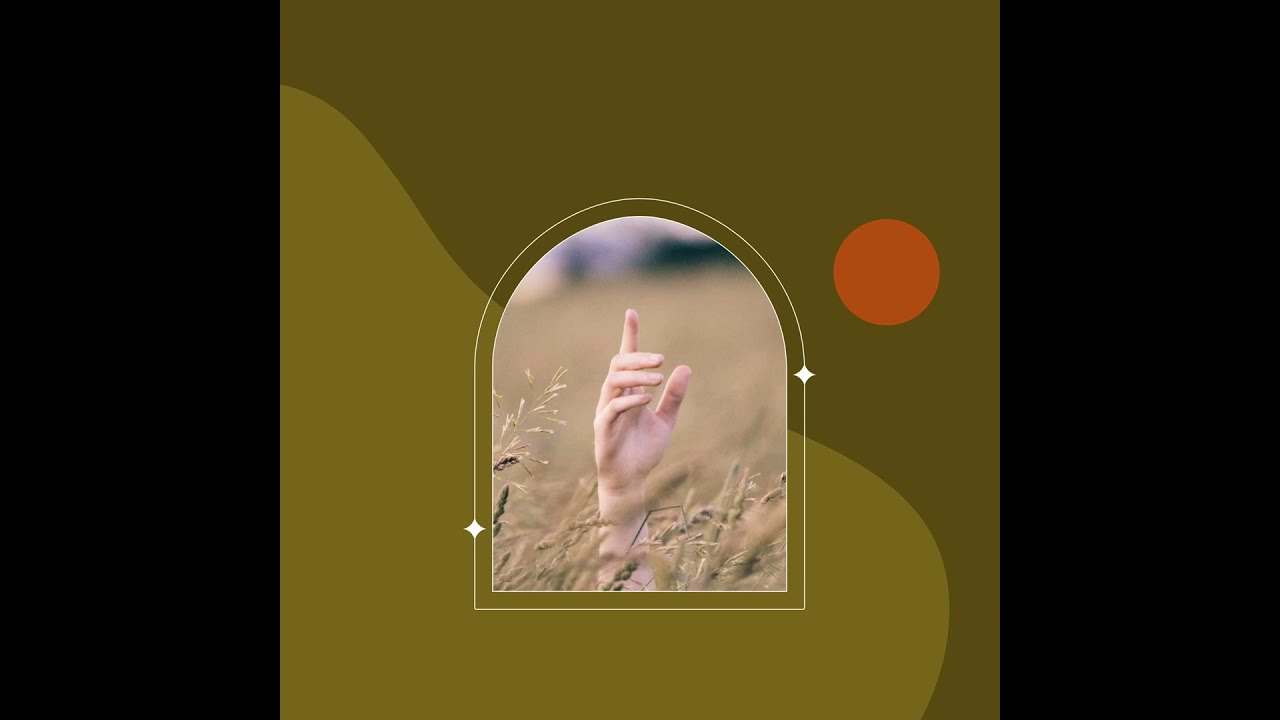The image features a widescreen layout bordered by black strips on either side, framing a central square. Within the square, there is a background comprising two olive green shades—dark green at the top and lighter green below—separated by a wavy line that curves from the upper left to the bottom right. In the darker segment, to the upper right, there's an orange dot. 

At the center of this green backdrop, an arch-shaped element with a white outline resembles a gravestone or memorial plaque. Inside this arch, a Caucasian hand emerges from a field of mostly yellow wheat, with hints of green. The hand's index finger points skyward, while the other fingers are slightly curled inward and the thumb curves upward and to the right. Small stars are positioned at the bottom left and upper right of the arched outline, adding a subtle decorative touch. This composition evokes a sense of both natural beauty and symbolic depth.